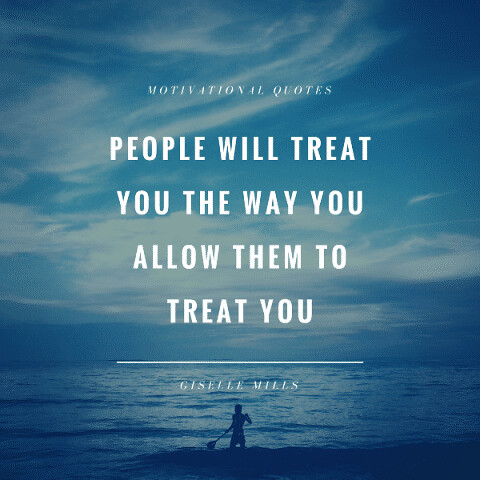The image is a digital poster displaying a motivational quote. The background features a serene evening ocean scene with a dark blue sea extending into the distance. The water has gentle waves and ripples, hinting at movement. Situated at the bottom of the image, silhouetted against the water, is a man either standing on the shore or on a small island, holding an oar or paddle. He appears to be looking out toward the sea, adding a contemplative mood to the scene. Wispy white clouds cover the top two-thirds of the image, giving it a hazy and tranquil appearance.

At the top of the poster, in very small letters, the words "Motivational Quotes" are written in uppercase white block letters. Centered on the image, in large uppercase white letters, is the motivational quote: "PEOPLE WILL TREAT YOU THE WAY YOU ALLOW THEM TO TREAT YOU." A thin white line underlines this quote, adding emphasis. Below this line, the name "Giselle Mills" is displayed in the same white uppercase letters, crediting the author of the quote. The overall composition of the poster is calming yet thought-provoking, effectively combining the visual elements with the powerful message.